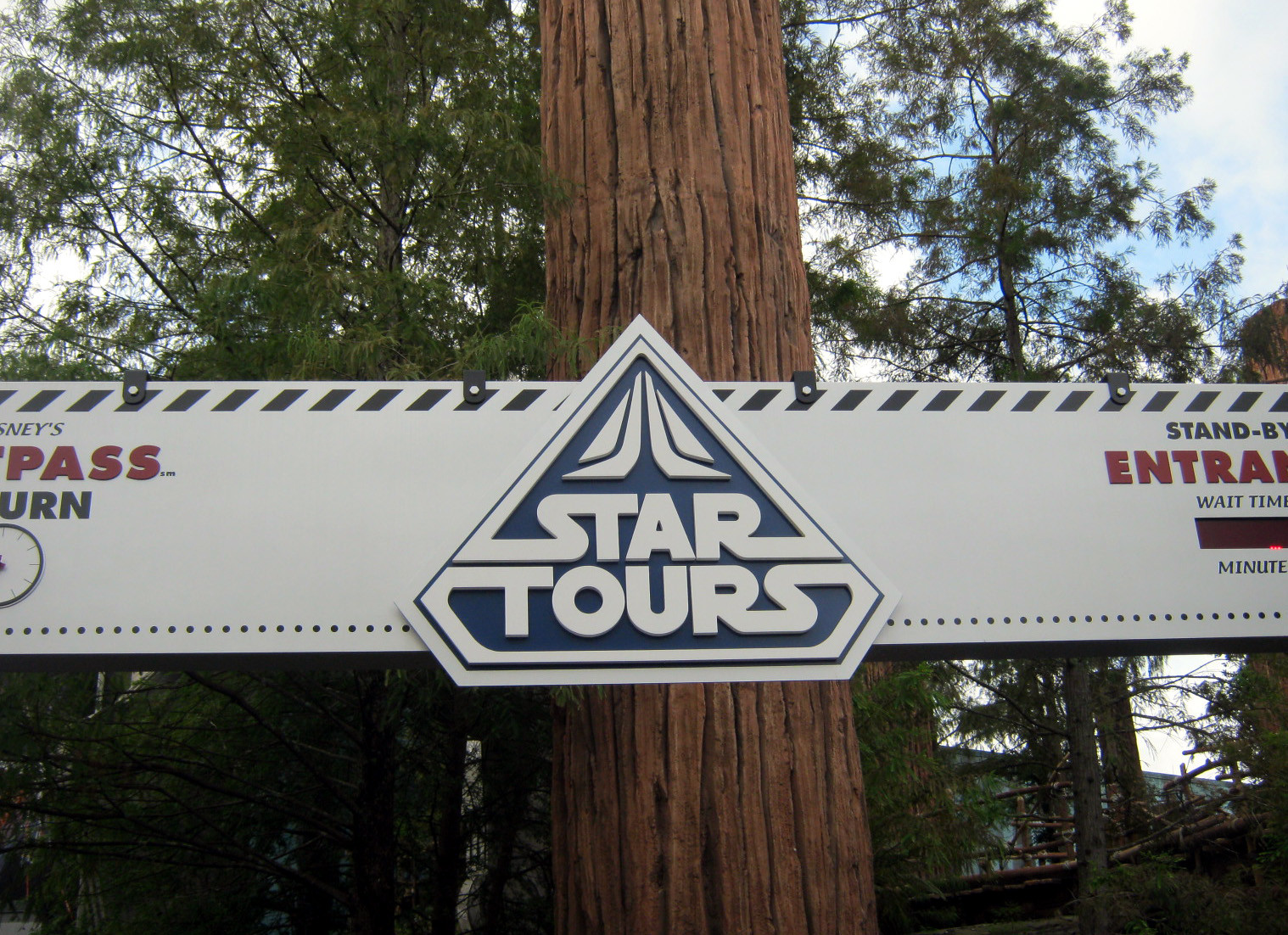The image depicts a detailed, color landscape photograph of an outdoor scene centered on a brown tree trunk with deep grooves. It is uncertain if the tree is real or an artificial replica. Surrounding the tree in the background are green-leaved trees and a clear blue sky. Horizontally affixed to the tree is a prominent white banner sign. In the middle of the banner is an upside-down diamond shape with a dark background and white lettering in the Star Wars font that reads "Star Tours." The top border of the banner features black rhombuses, while the bottom edge has black circles lining it. On the left side of the diamond shape, the banner appears to bear the partial word "Disney's" in white text, followed by red and blue information related to a Fast Pass. To the right side of the diamond, the sign indicates "Standby" in black letters, with the partial word "ENTRA" (likely part of "Entrance") in red letters underneath, followed by "Wait Time" and a blank area for time notation. The photograph captures the scene in vibrant detail, emphasizing the contrast between the structured sign and the natural foliage.